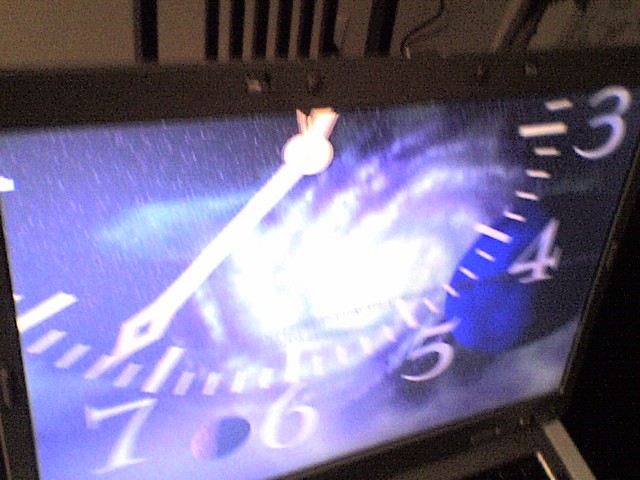The image is a close-up, taken from above, of a computer monitor or possibly a laptop screen, framed with a black plastic bezel. Dominating the screen is a detailed and colorful depiction of the lower half of a clock face. The clock's white minute hand is pointing a bit past the number 7. Visible numbers on the clock range from 3 to 7, each accompanied by smaller markers for each minute. The background of the clock face intricately blends a cosmic scene, featuring a vibrant spiral galaxy with a white core that fades into purplish and pinkish hues towards the edges. Scattered stars further embellish the scene. On the right side of the screen is a blue planet, while a purplish planet is situated at the bottom left. The surrounding environment includes a tan-colored wall intersected by vertical black stripes and a visible black cable extending from the monitor, suggesting that it is connected to another device. The edge of what appears to be a chair is faintly visible in the background.